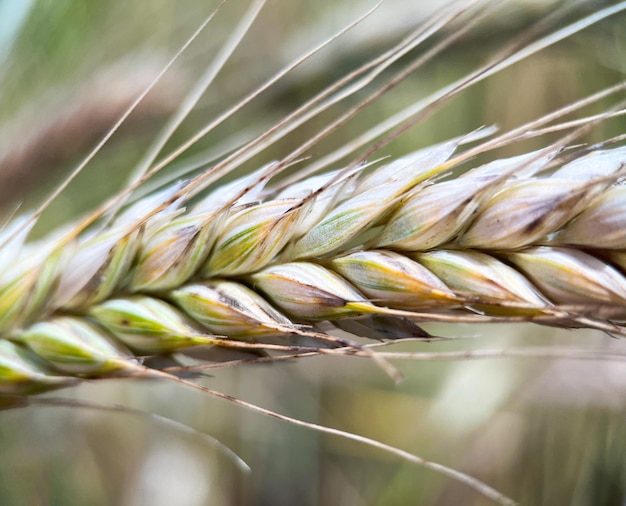The image captures a strikingly detailed, up-close macro photograph of what appears to be a sheaf of wheat, extending horizontally across the frame from the left center to the right center. The main stem, embedded with numerous oval, almond-shaped buds, is adorned with fine strands that stretch from the left center to various directions, some reaching the upper right and lower left corners. These buds are intricately layered, with muted yet richly interwoven colors of green, yellow, beige, and light brown, and tipped with darker brown hues. The background is beautifully blurred in a symphony of greens, yellows, blues, and purples, allowing the foreground's intricate details of the wheat to stand out. Each pod displays a gradient of colors transitioning fluidly, and thin, tan-colored strands extend delicately from them, highlighting the natural beauty and complexity of the wheat structure.